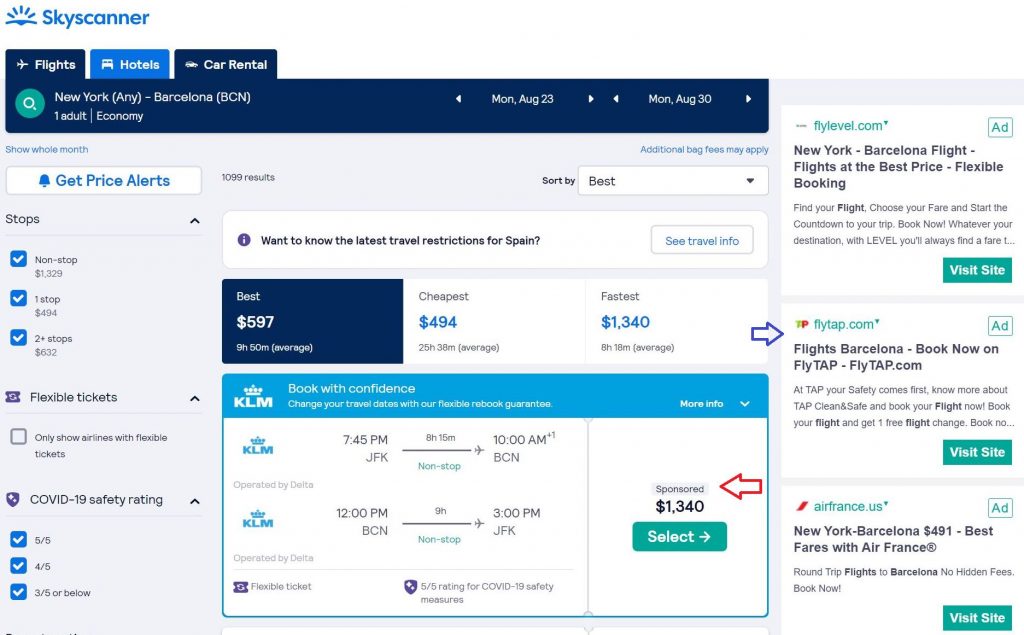This image showcases a webpage from a travel website, Skyscanner, designed for planning trips. At the top, there's a prominent white header featuring the Skyscanner logo in blue, with distinct blue lines forming a stylized horizon that ascend to the left and right. 

Just below the header is a dark blue navigation bar that spans about two-thirds of the page, containing various tabs to assist users in their travel planning. From left to right, these include a dark blue tab with a white airplane icon labeled "Flights," a light blue tab featuring a white hotel icon labeled "Hotels," and another dark blue tab with a white car icon labeled "Car Rental."

Underneath the navigation bar is a search section with a green search icon featuring a white magnifying glass. The search bar indicates a trip route from "New York NE" to "Barcelona BCN," with the travel dates listed to the right. Below this area, there are various filters and options including tabs for price alerts, non-stop flights, one-stop flights, two-stop flights, and COVID-19 restrictions.

On the right side of this section, a search bar appears with an adjacent tab titled "Want to Know for Travel Restrictions to Spain." Further down, a detailed pricing section is displayed with three categories: the best price, the cheapest option, and the fastest route, each highlighted in blue and white.

The central part of the page contains detailed flight information, including flight durations and prices listed on the right. Encasing this information is a white section bordered by a blue outline, which is thin along the sides and bottom but thicker along the top.

Running down the right side of the webpage, there are links to three additional websites, offering users further resources for their travel planning needs.